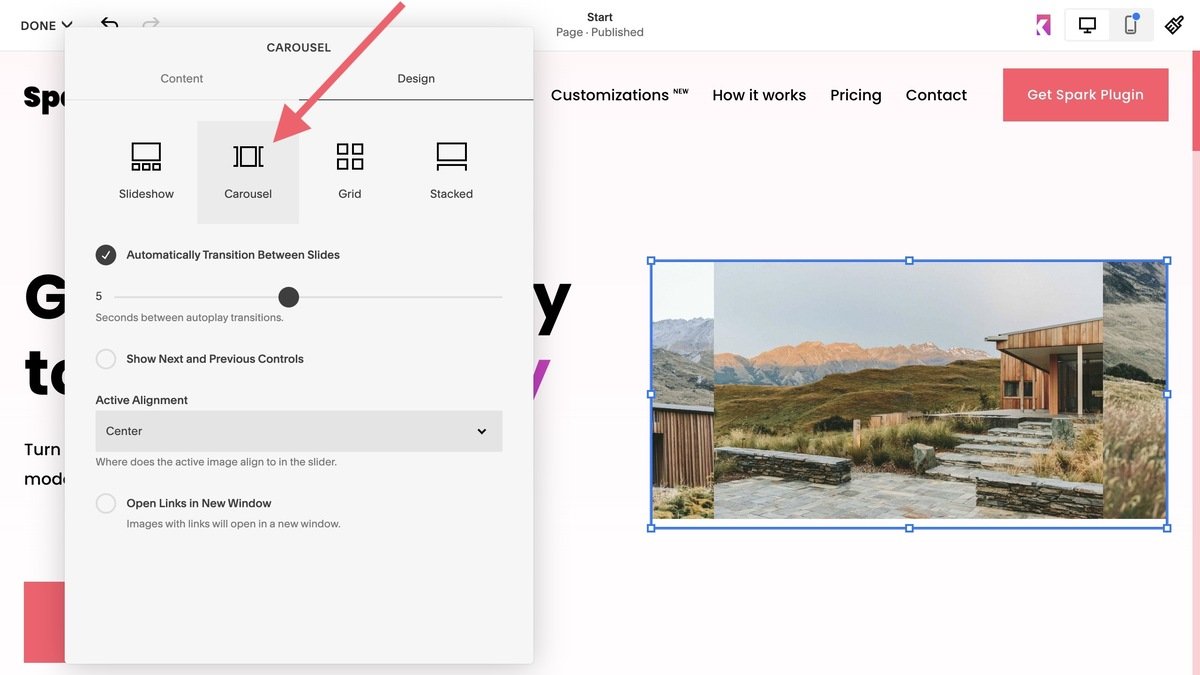**Descriptive Caption:**

The screenshot showcases a web page interface for cropping pictures.

At the top left corner, there is a "Done" button accompanied by a dropdown menu. Centrally located on the page, the word "Start" appears, followed by "Page" and "Published" underneath it.

In the upper right corner, four icons are displayed:
1. An icon resembling the right half of the letter 'K.'
2. An icon depicting a monitor.
3. A highlighted icon of a phone.
4. An icon that looks like a paintbrush.

An inset box partially obscures the name of the website and covers large text on the left half of the screen. This inset box, labeled "Carousel," offers two categories: 'Content' and 'Design.' The 'Design' category is highlighted with a black bar underneath it. 

Within the 'Design' section, users can select from four different options:
1. Slideshow
2. Carousel (highlighted by a red arrow)
3. Grid
4. Stacked

Below these options is the setting "Automatically transition between slides," which has been activated with a checkmark. A slider line, denoted with "5" on the left and adjusted to the middle, specifies the "Seconds between autoplay transitions."

Additional settings include:
- "Show next and previous controls," which is currently inactive (represented by a white circle with a grey border).
- "Active alignment," set to 'Center' with a dropdown menu, serving the function "Where does the active image align to in the slider."
- "Open links in new window," presently inactive, detailing that "Images with links will open in a new window."

On the top right of the screen, a prominent red button labeled "Get Spark Plugin" suggests 'Spark' might be the name of the website. Below this button is an image of a southwestern-style house featuring a stone-deck area, steps connecting the porch and driveway, with mountains visible in the sunlit background.

Surrounding the image is a cropping textbox outlined in blue, featuring white squares at the midpoints and corners of the lines for resizing.